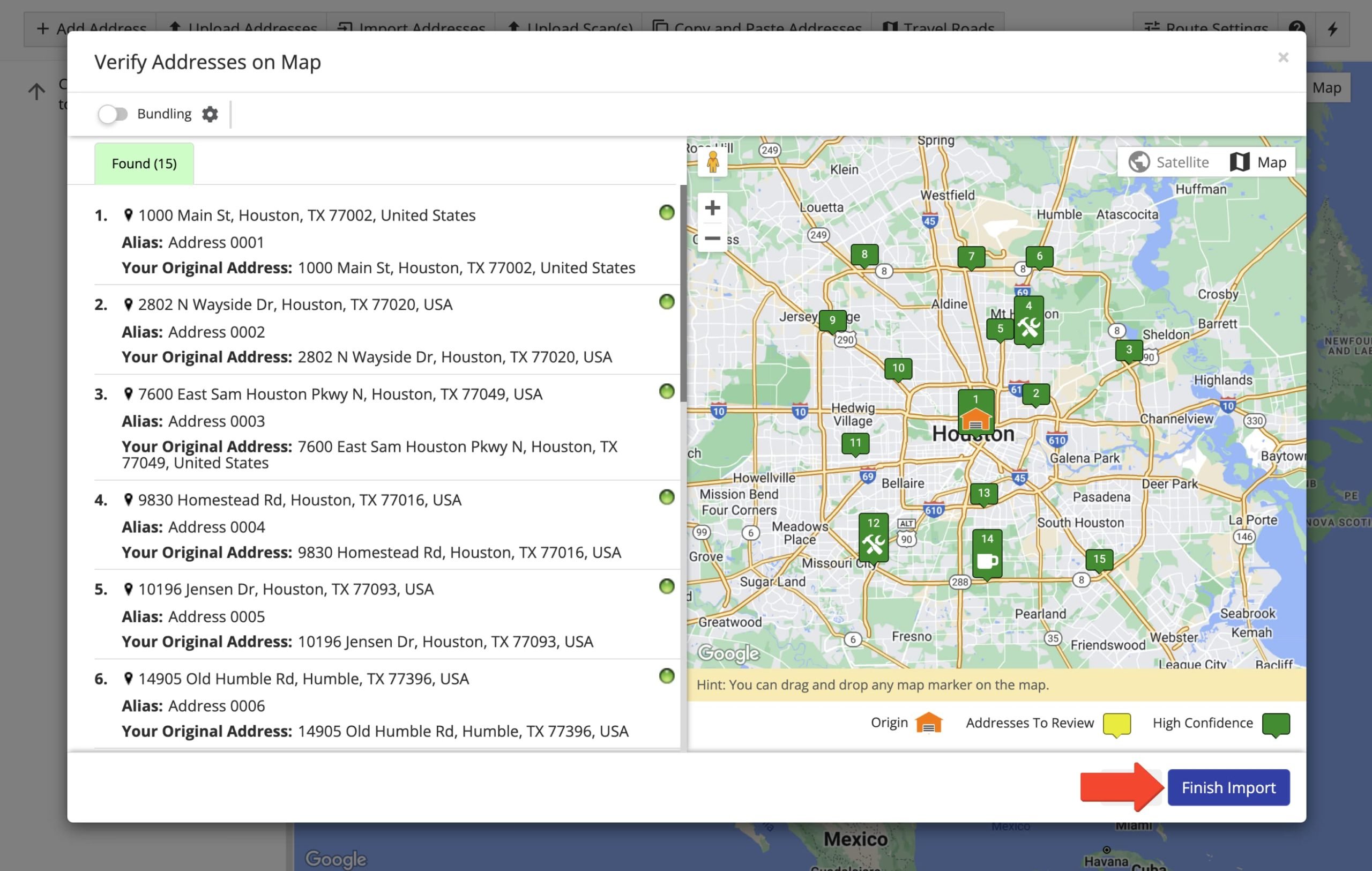An individual is diligently verifying addresses on a detailed map of Houston. The map features approximately 15 green box pinpoints scattered throughout the inner main part of the city. The very first pinpoint, prominently marked with an orange house icon, is located on Main Street, Houston, Texas. Each listing on the map displays both the current and original address, with six listings visible at a time and a total of 15 accessible via scrolling.

The user has access to both satellite and standard map views and can zoom in and out to examine specific areas closely. For a more immersive experience, the yellow human icon can be placed on the map to provide a street view. Several icons assist in navigation and identification: the orange house icon indicates the origin, a yellow chatterbox icon signifies addresses needing review, and a green chatterbox icon denotes addresses with high confidence.

Additionally, a helpful hint suggests that map markers can be dragged and dropped for more precise placement, augmenting the user’s mapping and verification tasks.